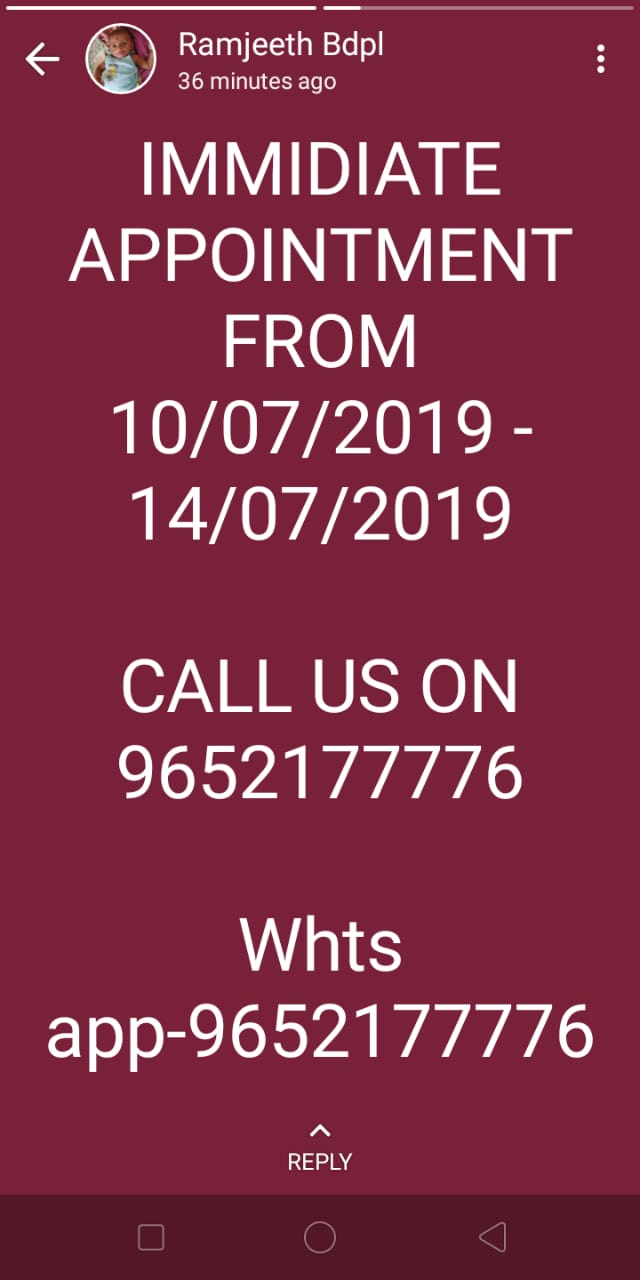This image is a screenshot from a cell phone displaying a social media reel with a rectangular shape, approximately 6 inches tall and 3 inches wide. The background is predominantly a deep burgundy color. At the top, there's a small circular photograph of a baby outlined in white, which is situated next to white text that reads "Ramjeet BDPL, 36 minutes ago." Below this, large white text announces "Immediate appointment from 10/07/2019 to 14/07/2019." Further down, it instructs viewers to "Call us on 9652 177776" and also provides a WhatsApp number formatted as "WHTS APP - 9652 177776." The screen also features a reply option with a white arrow pointing upwards. The footer of the image is maroon, featuring a white square, and on the left side, centrally located, is a white circle, while the right side has an arrow pointing left.